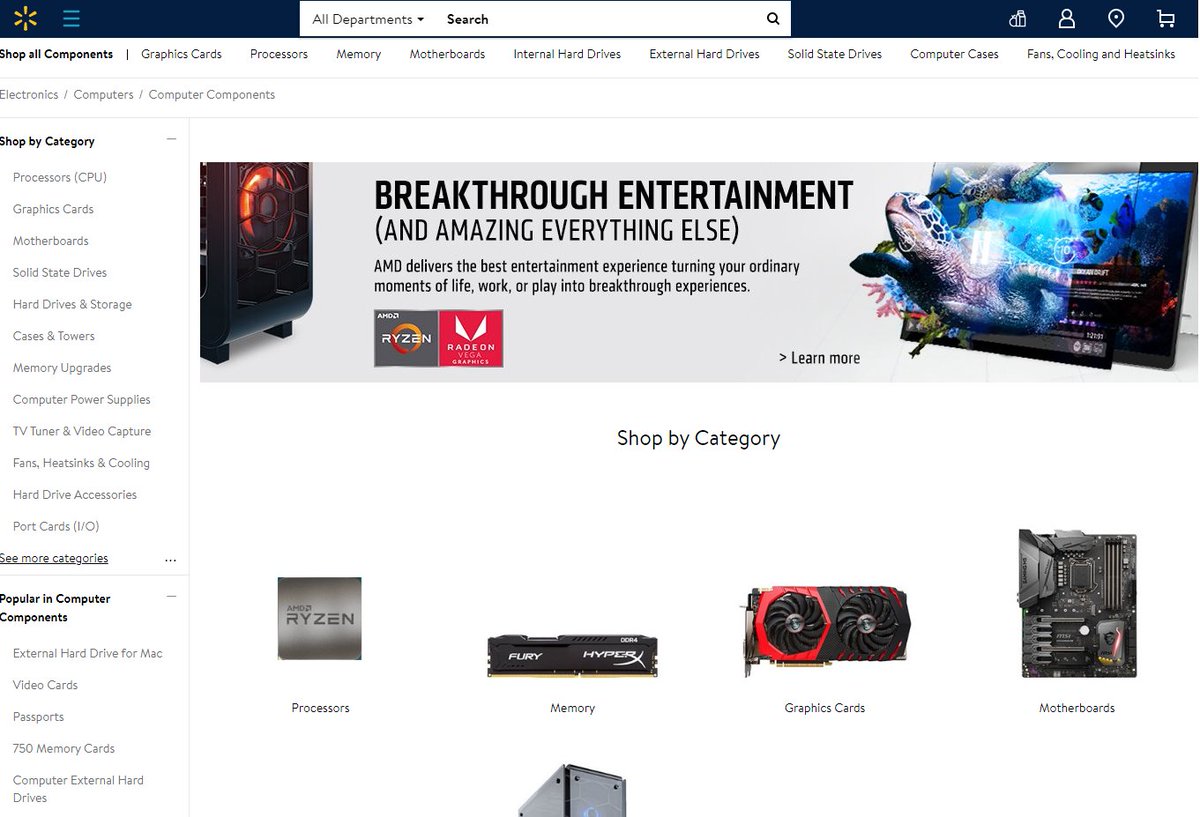This image, sourced from a web page, showcases the Walmart website. At the top, the distinct Walmart logo—six yellow petals arranged in a circular pattern resembling a flower—is prominently displayed. Just beneath the logo, navigation options are visible, including an "All Departments" dropdown menu and a search bar for browsing various items.

The main focus of the page features a promotion for AMD products. On the left side, a heater is partially visible, while on the right, a TV or computer screen displays a dynamic image of a turtle and other sea life emerging from the screen. This eye-catching visual is accompanied by the text "Breakthrough Entertainment and Amazing Everything Else," underscoring AMD’s promise of an exceptional entertainment experience. The caption elaborates that AMD technology transforms everyday moments—whether for life, work, or play—into extraordinary experiences.

Below this main section, the page is divided into categories for easy navigation, encouraging users to "Shop by Category." Images and links for various components are visible, including processors specifically branded as Ryzen, memory, graphics cards, and motherboards. Unfortunately, the image cuts off, preventing further details from being seen.